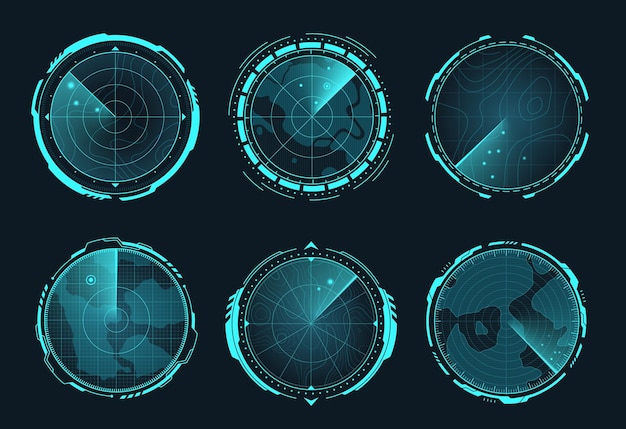This landscape-oriented image, possibly digitally generated, presents six radars or meters, each with unique designs, set against a bluish-black background. Organized in two rows of three, these scopes feature an illuminated bright aqua rim and intricate interior patterns. The patterns vary from cartographic and spiral designs to water-themed backgrounds, each interspersed with radar-like elements such as circles, lines, pins, and dots indicating various detections. As the radar lines sweep across their respective dials, sections briefly illuminate in bright blue, highlighting different quadrants and shapes. The composite detail and the variety in the scopes suggest they might be detecting movement or navigating, invoking sensations of exploratory technologies such as those used in submarines, airplanes, or terrain mapping. Each radar appears to be actively scanning, adding a dynamic, animated feel to the intricate and visually engaging composition.